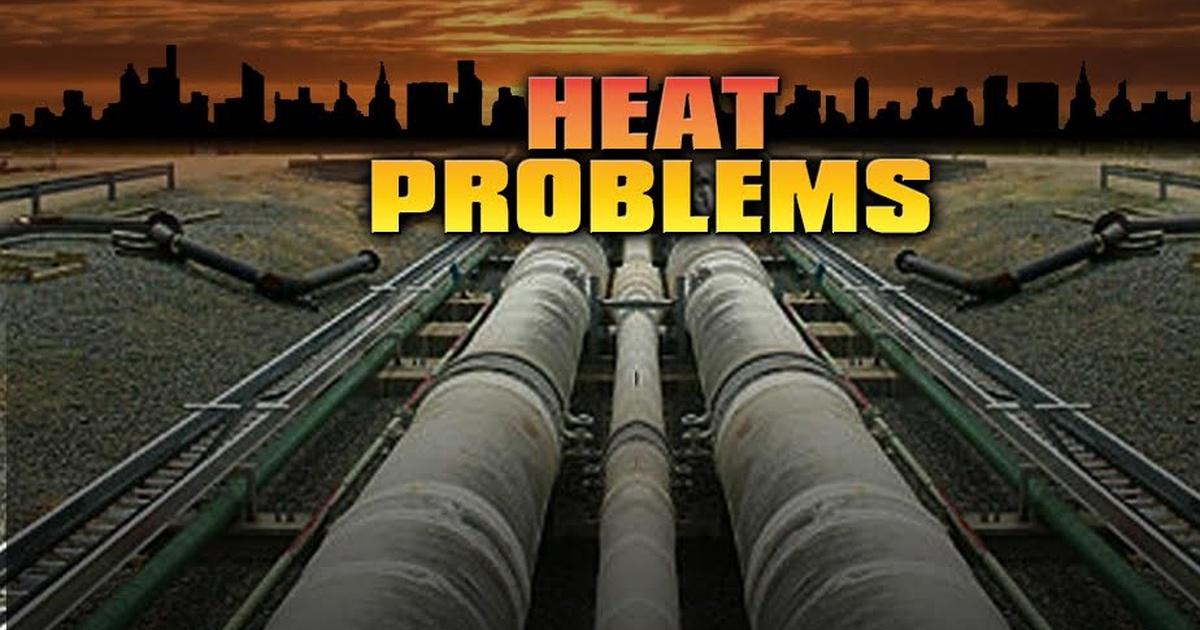The image is a low-resolution poster depicting the top of a building with prominent external air ducts and large pipes, possibly made of metal. The scene captures a silhouetted chocolate brown city skyline in the far distance, set against a striking backdrop of a sunset sky, displaying hues of light orange, yellow, rust brown, and sepia. The text "HEAT PROBLEMS" is emblazoned across the upper part of the image in capitalized letters, featuring a gradient from orange to yellow for the word "HEAT" and transitioning to solid yellow for "PROBLEMS." The ventilation equipment, characterized by gray and slightly greenish tones, is centrally featured, flanked by beveled areas with hook-like designs hanging towards the lighter-colored tubes. The photograph, presented in a wide-angle format with a shallow vertical length, emphasizes the theme of urban heat management under the intense sunset glow.